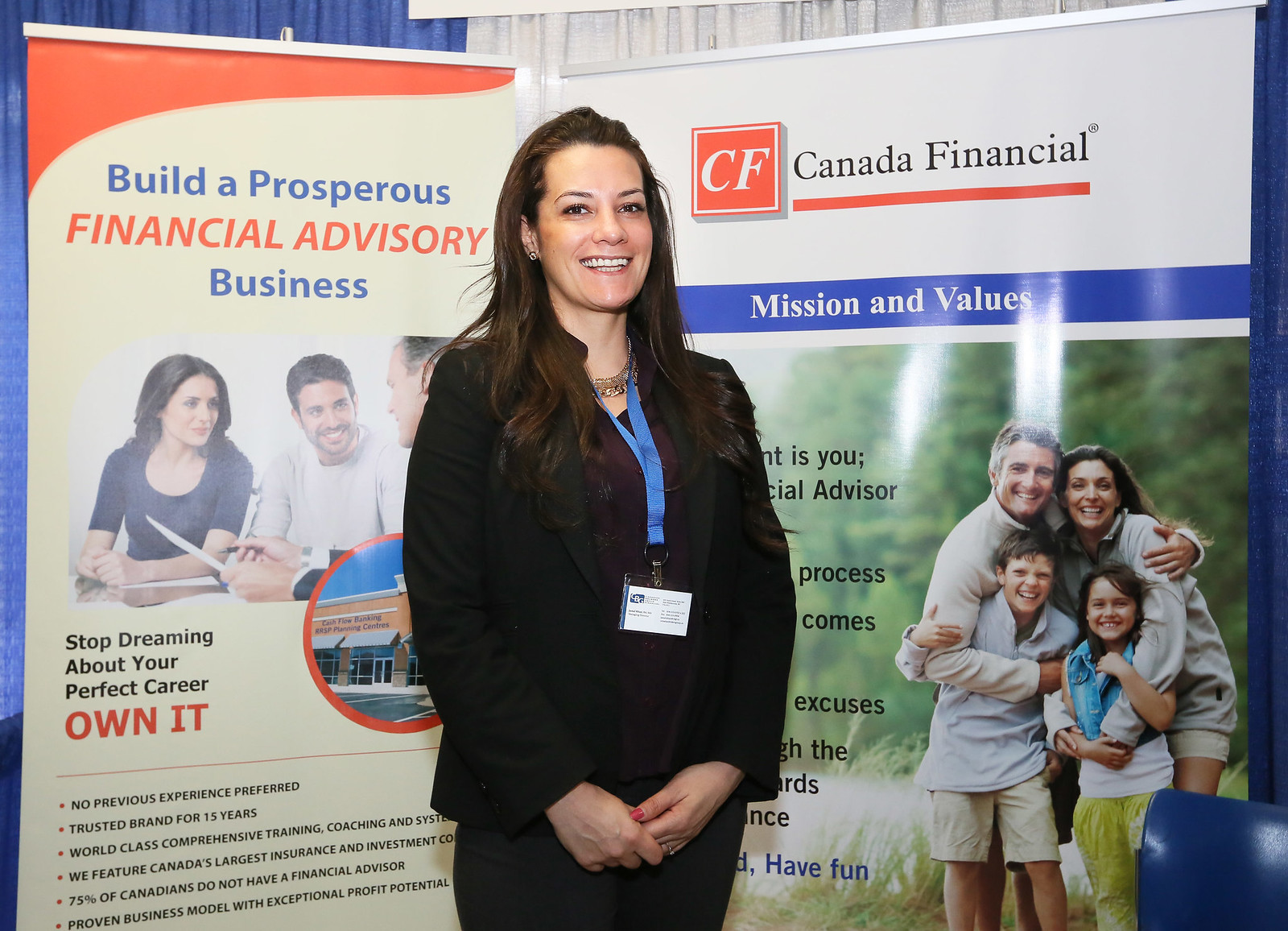In this image, a woman stands confidently while smiling at the camera. She is dressed in a black jacket over a blue shirt, accessorized with red nail polish, earrings, and a golden necklace. A blue lanyard with a white ID card hangs around her neck. Her dark brown hair frames her face as she stands in front of two distinct posters. The poster on the left features a white background with blue and red text that reads, "Build a prosperous financial advisory business." It includes images of three individuals: a female on the left and two males on the right, with additional text below that stating, "Stop dreaming about your perfect career." The poster on the right promotes "Canada Financial Business and Value." The overall scene suggests a professional setting, likely related to financial advisory services.